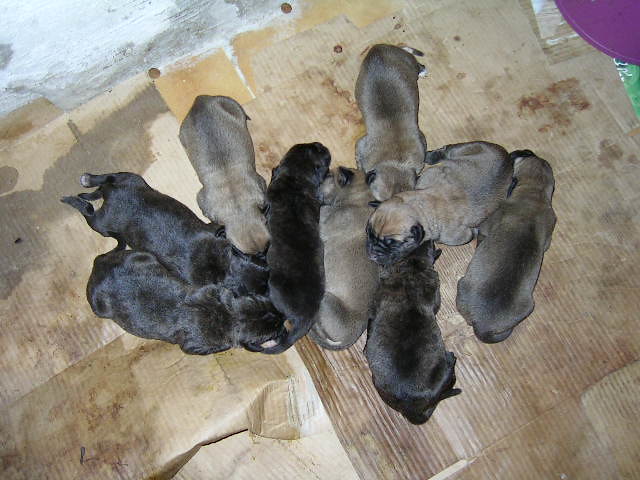The photograph captures a litter of approximately eight to nine newborn puppies, likely of a bulldog breed, sleeping huddled together on a makeshift bedding of stained, corrugated cardboard pieces that appear old and worn. The puppies are a mix of black and light brown coloration, with a few black ones situated near the center, forming a loose 'V' shape configuration. Their bodies are intertwined in a haphazard manner, with some resting their heads atop others, all connected in a close, shared sleeping space. The scene is further framed by a partial view of a purple circular object in the upper right-hand corner and a glimpse of a concrete wall in the upper left-hand portion of the image. The background also reveals bits of a linoleum floor, reinforcing the impression that this is a temporary setup designed for the comfort and care of the puppies.